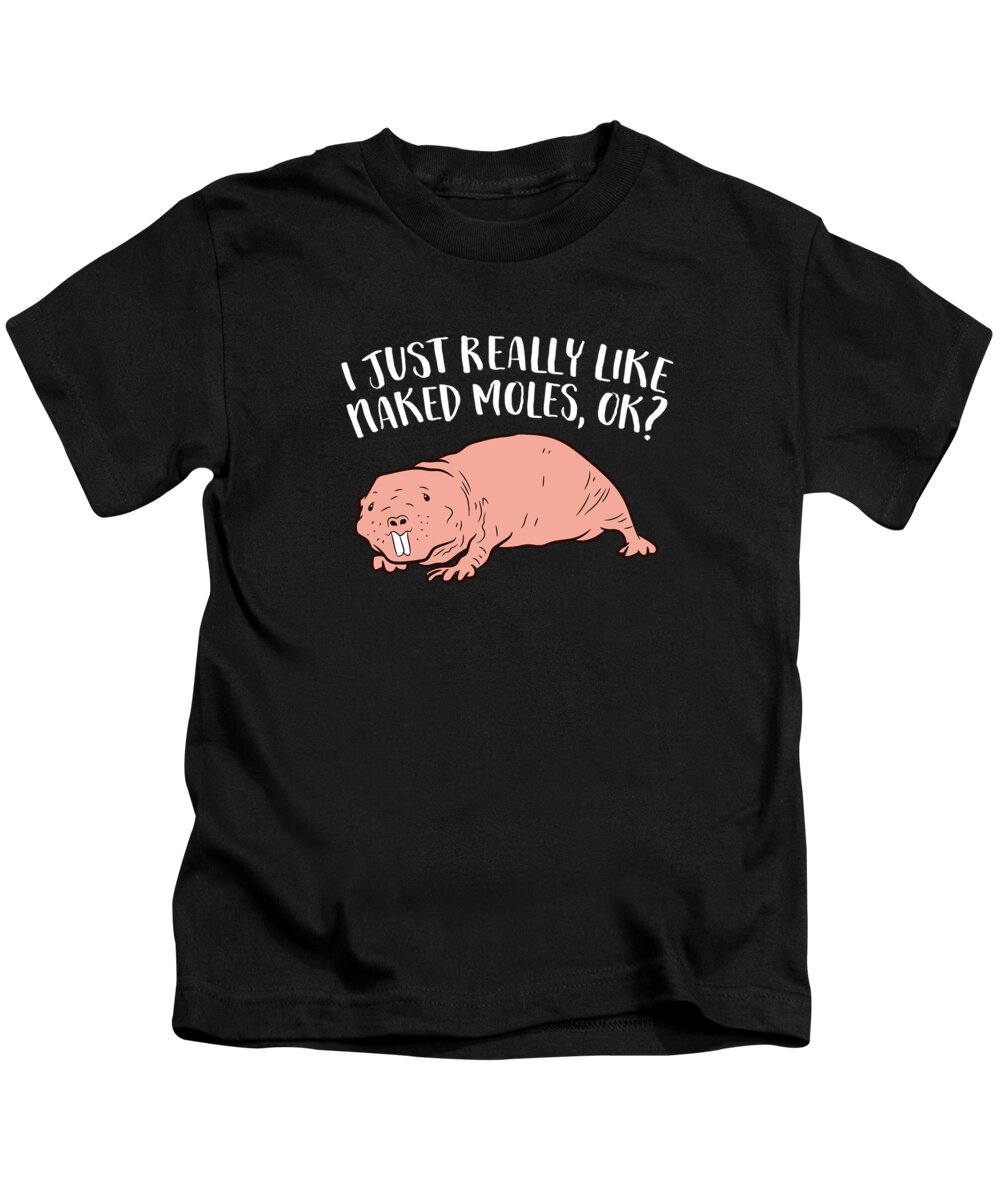This image shows a black, short-sleeved t-shirt featuring a comedic design. The upper part of the shirt displays the humorous white text: "I just really like naked moles, okay?" styled in a slightly arched formation. Below the text is a cartoon-like drawing of a bright pink mole with two prominent buck teeth, black eyes, and nostrils. The mole, depicted with thin black lines to suggest wrinkles and faint dots implying whiskers, appears to be looking at the viewer. Positioned side-on, the illustration reveals three of its four legs, with one front paw and a back foot visible. The t-shirt is clearly meant to be humorous, potentially for advertisement purposes.